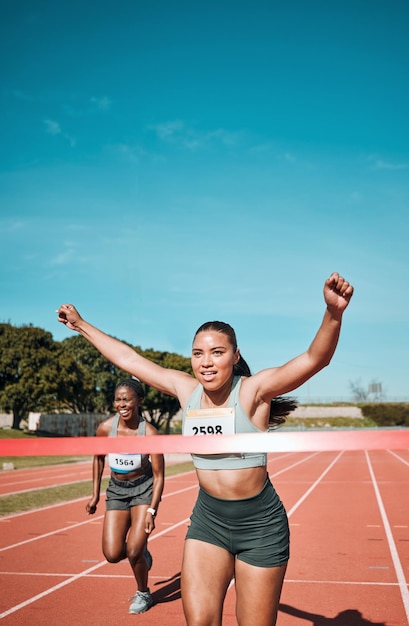In this vibrant outdoor daytime photograph, two black women are captured in a thrilling moment of a race. The scene unfolds on an orange-colored racetrack with distinct white markings, under a striking ocean-blue sky. The track consists of six lanes and is flanked by lush green trees, and possibly, a gray stone wall or terrace with some bushes in the background.

The focal point of the image is the leading runner, poised to break through the peach-colored finish line tape stretched across the lower third of the picture. She exudes triumph, her arms raised victoriously in the air. She sports a gray midriff-baring tank top, prominently displaying the number 25981, paired with green shorts. Her joyful smile and energetic wave amplify the exhilarating moment.

Trailing slightly behind her is another black woman, dressed identically in a gray tank top and green shorts. Her race number, 1564, is clearly visible. She too is smiling, radiating the contagious excitement of the competition.

The photo beautifully captures the essence of victory and the spirited camaraderie of the race, set against a picturesque, sunny backdrop.